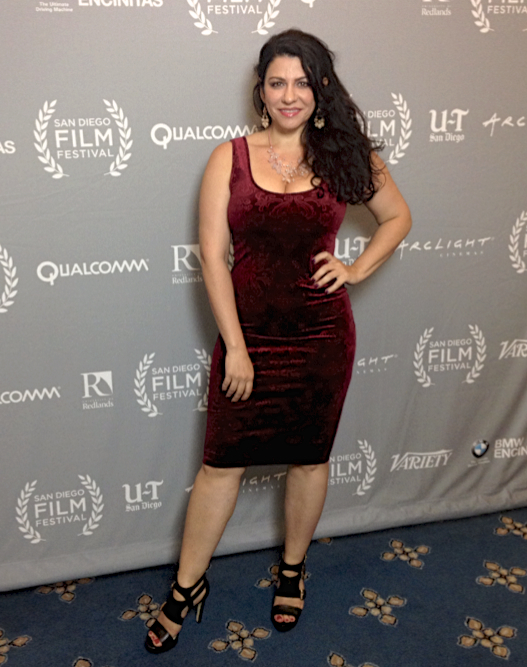In this color photograph, a striking woman, likely in her late 20s to mid-30s, is standing on a dark blue carpet adorned with gold diamond shapes at what appears to be a red carpet event. She is wearing a captivating red velvet dress that falls just above her knees. The dress is sleeveless with tank top straps, highlighting her black hair, which is styled to fall over her right shoulder while being tucked back on the left. Her accessories include black high-heeled sandals, a diamond necklace, and gold earrings, adding a touch of elegance to her ensemble.

She stands confidently with her left hand placed on her hip, looking up at the camera with a radiant smile. The backdrop behind her is a gray banner wall covered in logos, including "San Diego Film Festival" in prominent white type accented by white wreaths on either side, and other sponsor names like Qualcomm, Variety, BMW, and U/T San Diego. The overall ambiance captures the glamour and excitement of the event, suggesting she could be an actress or notable talent attending the San Diego Film Festival.